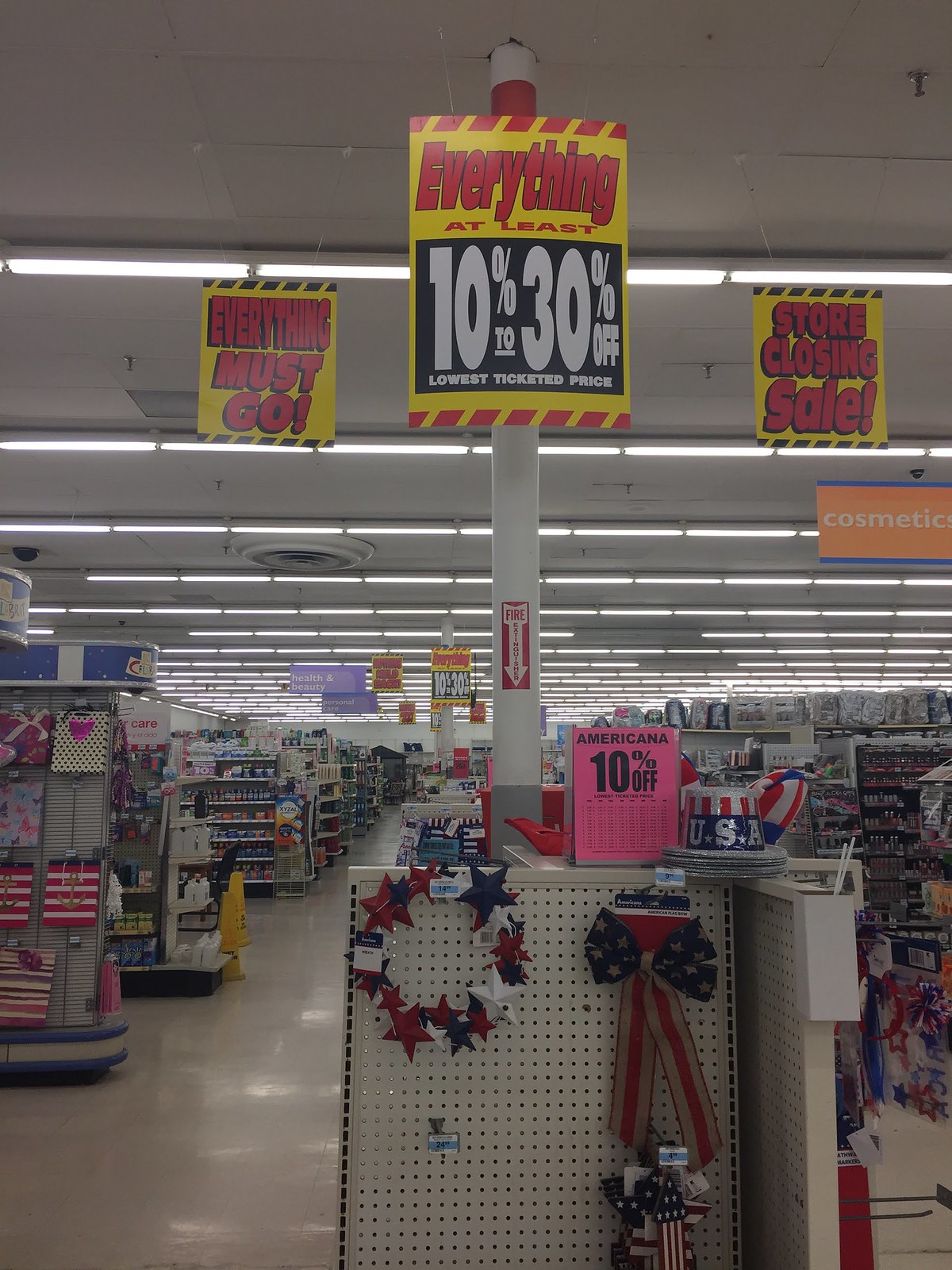This photograph captures the bustling interior of a shopping center, with a particular stand taking center stage. Dominating the stand is a pole extending from floor to ceiling, adorned with a paper sign. This sign draws the eye with its bold, red lettering on a yellow background proclaiming, "Everything." Below, in smaller text, it states "at least," leading to a black, slightly rectangular box with white text that announces "10% to 30% off." Completing the message, the phrase "lowest ticketed price" is neatly printed underneath.

The ceiling above is composed of white, rectangular acoustic tiles, from which several fire safety sprinklers protrude, including a prominently visible one in the top-right corner. The ceiling is illuminated by rows of horizontal fluorescent lights stretching from the foreground to the back of the image.

The image provides a sense of depth with aisles visible on the left and right, beginning about a third of the way from the respective edges and disappearing out of the frame. These aisles are lined with various products.

The display stand is festooned with USA-themed items. On the top right of the stand rest small, glittering silver USA hats. The front of the stand features a pegboard, painted white, with numerous hooks for hanging displays. Attached to this pegboard is a wreath-like circle composed of stars in red, blue, and white. To the right of this, a blue ribbon decorated with white stars hangs elegantly next to a ribbon adorned with red and white stripes. The overall scene is vibrant, indicative of a lively shopping environment celebrating USA-themed merchandise.